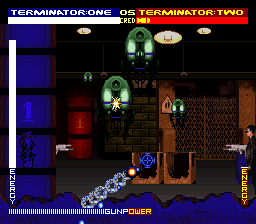This is a detailed screenshot from a shooter video game featuring a character reminiscent of the Terminator. At the top left-hand corner of the screen, the white text "Terminator 1" is displayed over a blue background, accompanied by a large white health bar underneath. On the right-hand side, "Terminator 2" is written in yellow with a red background and has a health bar below it, which is mostly red with a small sliver of yellow. The screen predominantly features colors like blue, red, and brown, giving the impression of a warehouse setting with blue walls and a gray floor.

In the bottom right-hand corner is a character resembling the Terminator, facing left. This character has a black jacket, black sunglasses, and dark hair, and is holding and aiming a large silver gun to the left. Above the character, the word "Energy" is written vertically in yellow, on a red background. On the screen’s left side, there is a vertical display with the word "Energy" in white, and a white bar above it. Below this is another meter labeled "Gun Power," divided into white and yellow segments.

Additionally, there are targets seen floating up in the sky, which vary in color, including blue and green. A blue reticle indicating the gun's aiming point is visible on the screen, hinting at active shooting mechanics. Overall, this screenshot captures an intense, action-packed moment from the game, with numerous game mechanics and status indicators overlaid on the scene.